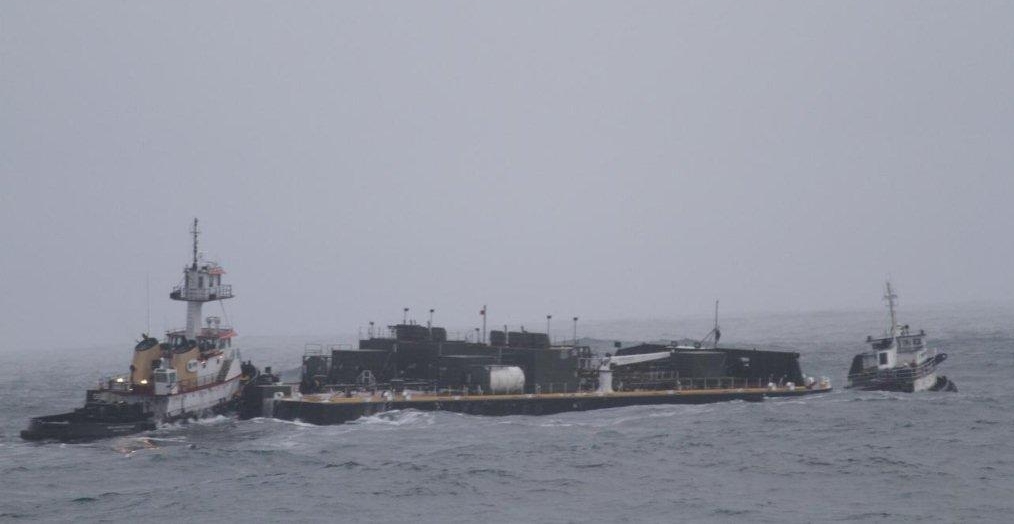In this image, three vessels navigate through choppy, gray waters under a cloudy sky, creating a low-contrast scene with murky hues. At the center is a large black cargo ship or barge with a brown deck that appears to be carrying railroad cars. To its left, a smaller vessel with its lights on seems to be assisting, possibly towing the barge. It has an elevated lookout area. Behind the barge, a third, larger boat follows, featuring multiple circular structures and appearing to monitor or assist the barge. The overall atmosphere is one of rough seas and overcast skies, enhancing the sense of a challenging maritime endeavor.